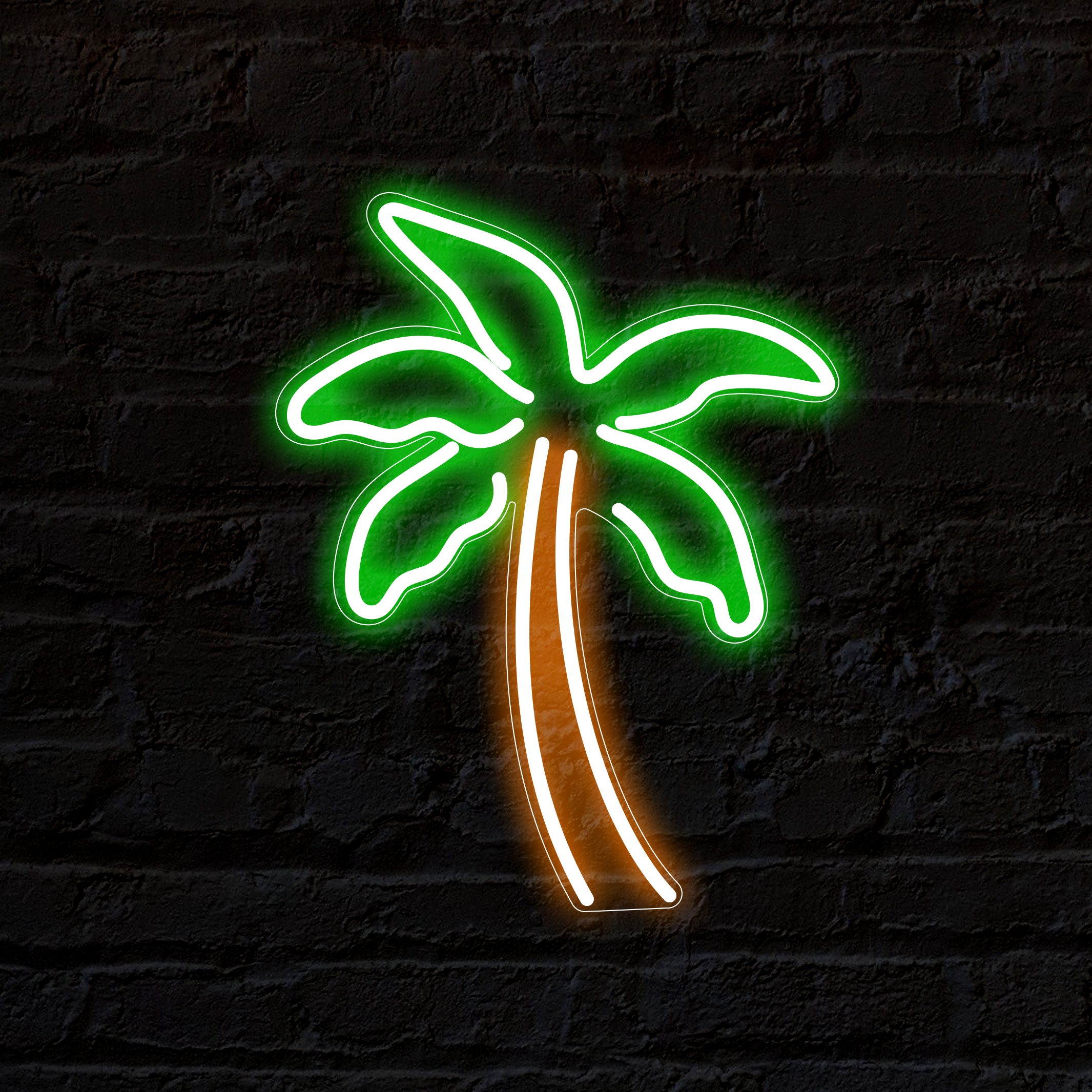Against a dark black, textured brick wall, painted nearly chalk-black to accentuate its details, hangs a striking neon sign of a palm tree. The palm tree's five vivid neon green fronds — three upwards on the left, two angled downwards on the right — illuminate brightly against the brick background. The trunk features two neon lights, curving slightly to create a lean, and emits a glowing brown hue that completes the lifelike appearance. The rough, ridged wall enhances the image, providing a perfect contrast to the vibrant neon details of the palm tree set in the middle of the photo.